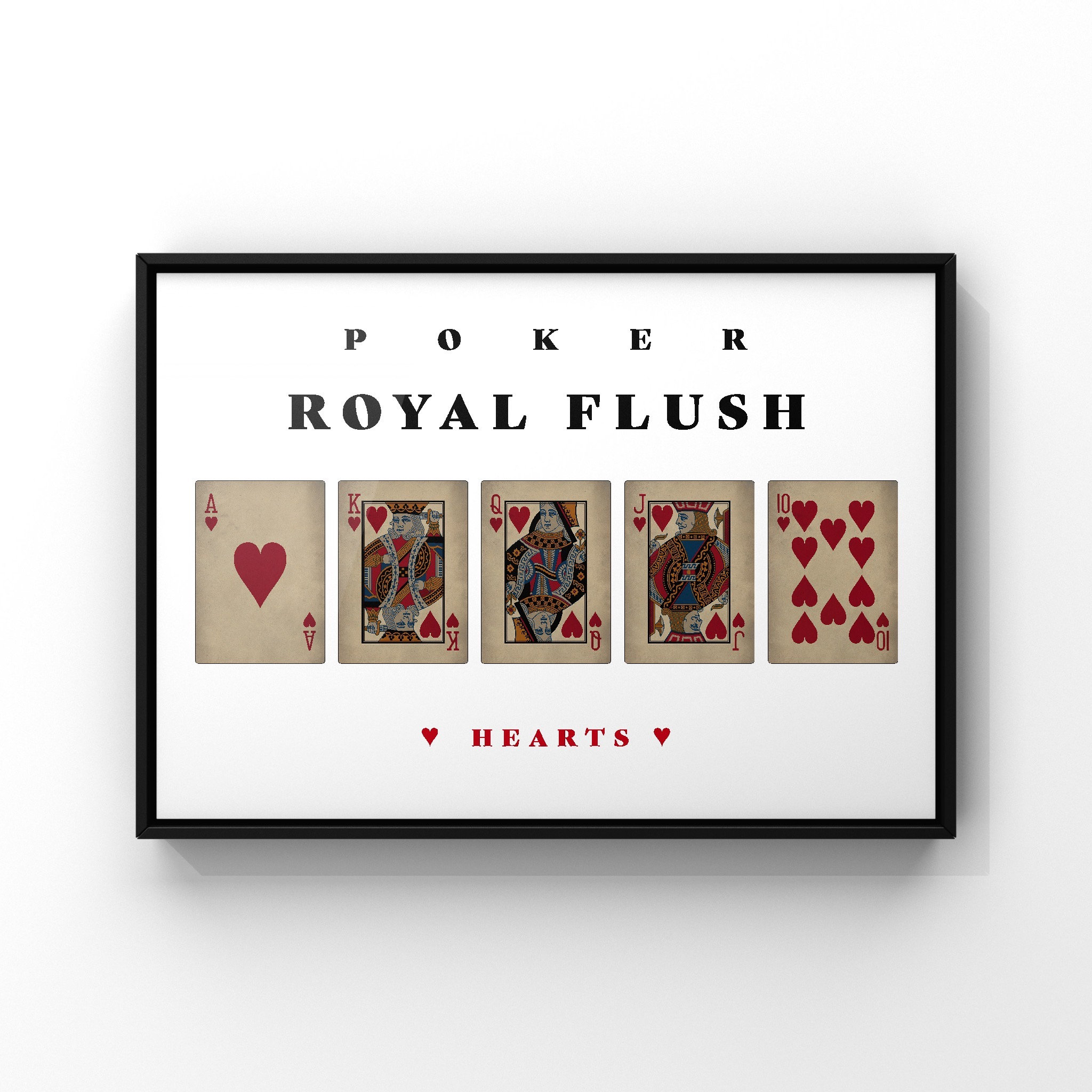The image features a framed art piece with a black frame against a white background, casting a shadow that suggests it is hung on a wall. Inside the black frame, there is a white backdrop with the word "Poker" inscribed at the top in black letters, followed by the phrase "Royal Flush." Below this text, there are five playing cards arranged sequentially: the Ace of Hearts, King of Hearts, Queen of Hearts, Jack of Hearts, and Ten of Hearts, all depicted with a simplistic, somewhat worn design. Below the cards, the word "hearts" is written in bold red letters, flanked by two red heart graphics. The overall presentation of the cards and text captures the essence of a Royal Flush in the hearts suit, creating a striking visual representation suitable for wall decoration.